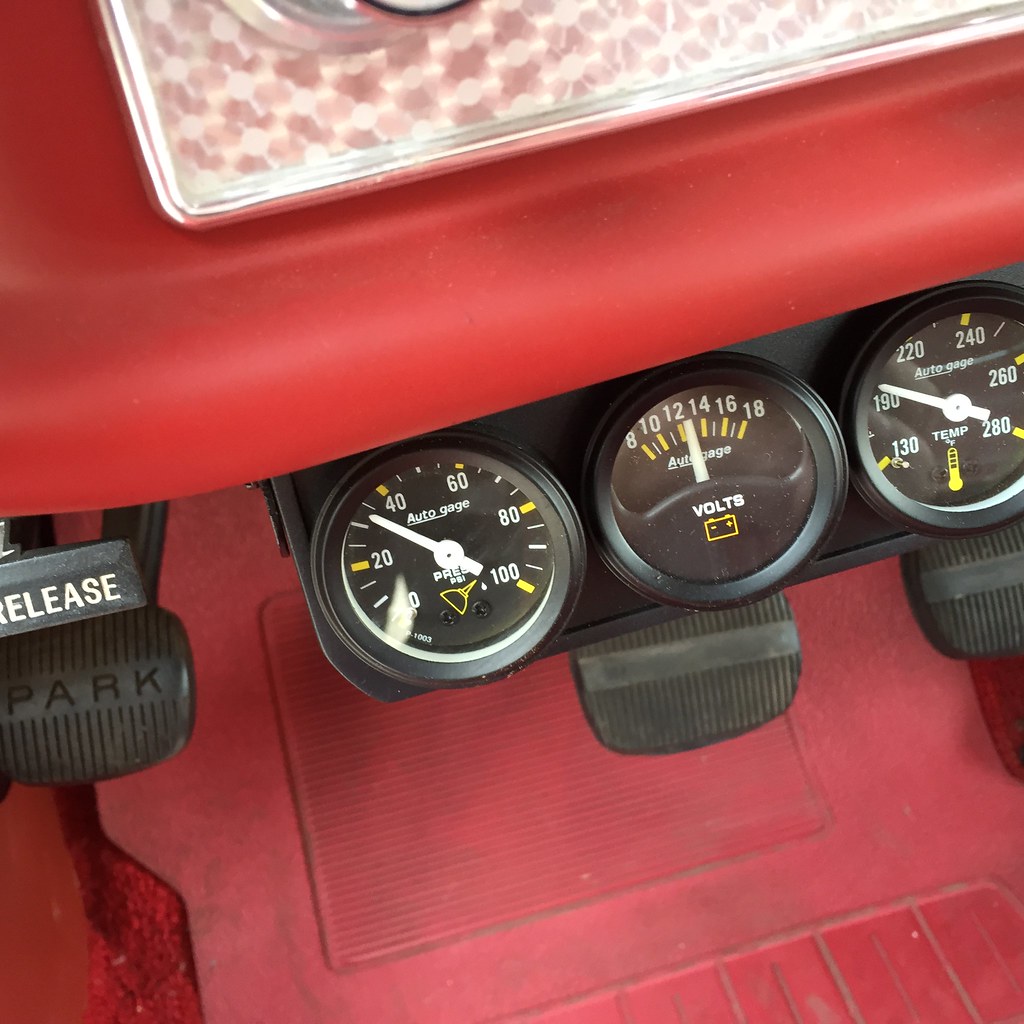The image depicts the interior of a vintage car, focusing on the dashboard and floor area. Dominating the red dashboard are three black gauges with silver bezels, positioned centrally in the image. From left to right, the first gauge measures oil pressure in psi, indicating just under 35. The next gauge measures volts, showing around 13 volts between the 12 and 14 marks. The far-right gauge measures temperature, reading just over 190 degrees Fahrenheit. Below these gauges, we can see the red rubber floor mat with red carpeting peeking out beneath, accompanied by black pedals including a gas pedal and a parking brake with a release lever. The overall color scheme features red, black, and silver, reinforcing the vintage aesthetic of the car interior.